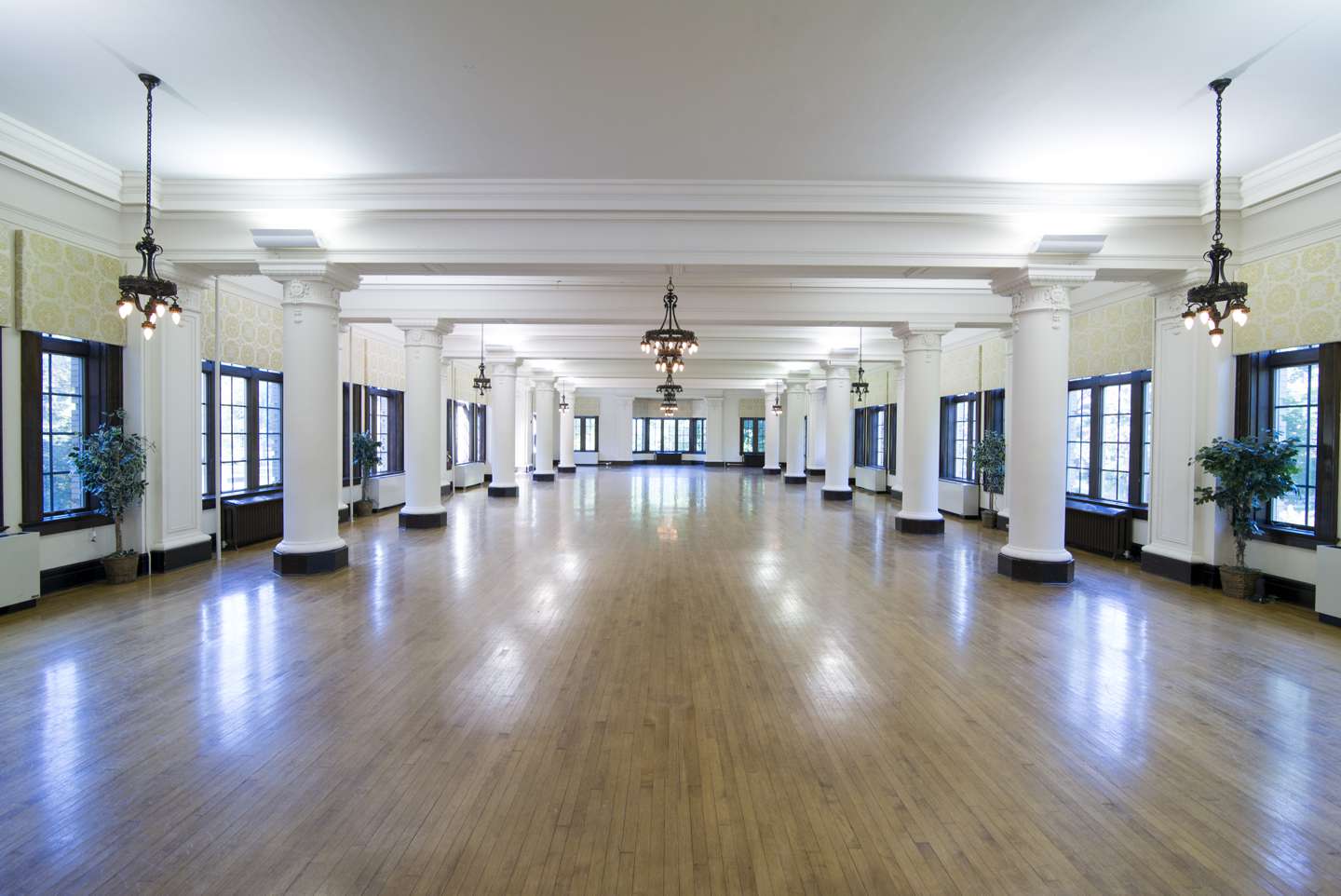The image captures an expansive and empty hall with polished pine wood floors that reflect the incoming light from numerous windows lining both sides of the room. The gleaming reflections also showcase light from multiple chandeliers hanging symmetrically from the ceiling. The chandeliers vary, with larger ones in the center and smaller, but similarly styled black chandeliers towards the sides. The hall's ceiling is supported by several white columns, and white beams stretch across the ceiling. The walls, painted in white with intricate flowery pale yellow or cream patterns at the upper sections, add a touch of elegance. Additionally, there are large green potted plants, resembling ficus trees, positioned beside the windows. The room's symmetry and details, such as the mix of white and beige tones and the presence of box-like structures by some of the windows, contribute to an impression of it possibly being a dance hall, accentuated by a large bay window at one end of the room.